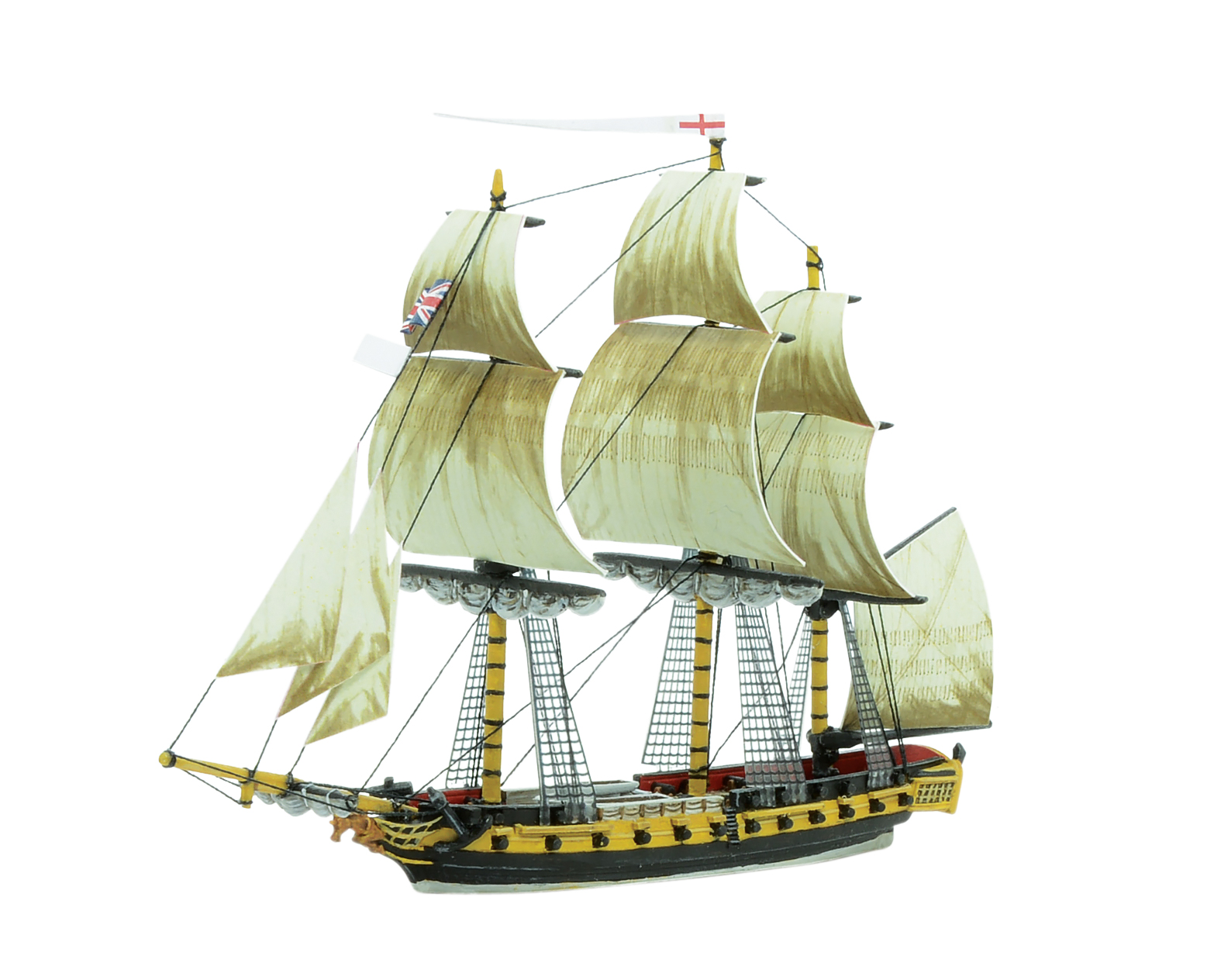The image depicts a detailed drawing of an ancient, vintage sailboat with a pirate ship-like appearance, set against a plain, white background. This tall ship features a black hull with a yellow band running along the top edge. The structure includes three masts, each adorned with long white flags bearing a red cross. The ship flaunts multiple sails, varying in size and color from pale green to light brown, with some billowing and others neatly drawn up. A red interior can be seen, resembling teak wood, while networks of ropes, resembling nets and checkerboards, intricately criss-cross from the hull to the sails. Cannons line the beige wooden deck, adding to its warship aesthetic. The front of the ship, pointing left, displays some barely legible letters on the yellow band. The sails and details make it look like an incredibly realistic toy or model rather than a real historical vessel.